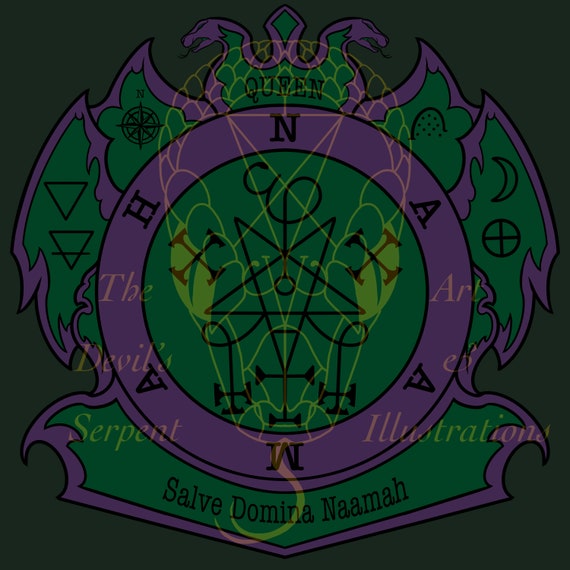This digitally drawn logo features a solid muddy greenish-black background, overlaid with intricate and ominous details that suggest a dark, possibly religious symbolism. At the center of the logo, a dark green circle is enclosed by a thicker, vibrant purple ring inscribed with the letters "H N A A M A." Above this central circle, there are two pink serpent heads facing outward, crowned with a small star-like symbol.

Encircling the green and purple core, are wing-like structures with jagged, uneven edges, giving a sense of movement and aggression. Upon closer inspection, faint lime-green lines form the subtle outline of a snake head and scales, with the snake's tongue ominously flicking outwards.

At the top of the design, a crown and the word "Queen" are prominently written in black letters, flanked by images of serpent heads. Along the perimeter of the purple ring, a variety of symbols appear, including a compass, inverted crosses, and iron crosses. 

The bottom section of the logo is supported by a wider, curved base, also exhibiting green and purple tones. This base contains the banner "Salve Domina Nama," intertwined with dark, curling lines and additional symbols like an inverted five-pointed star, triangles, and crescent moons. Faint yellow text phrases like "the devil's serpent" and "art of illustrations" are scattered around the design, further emphasizing its sinister theme.